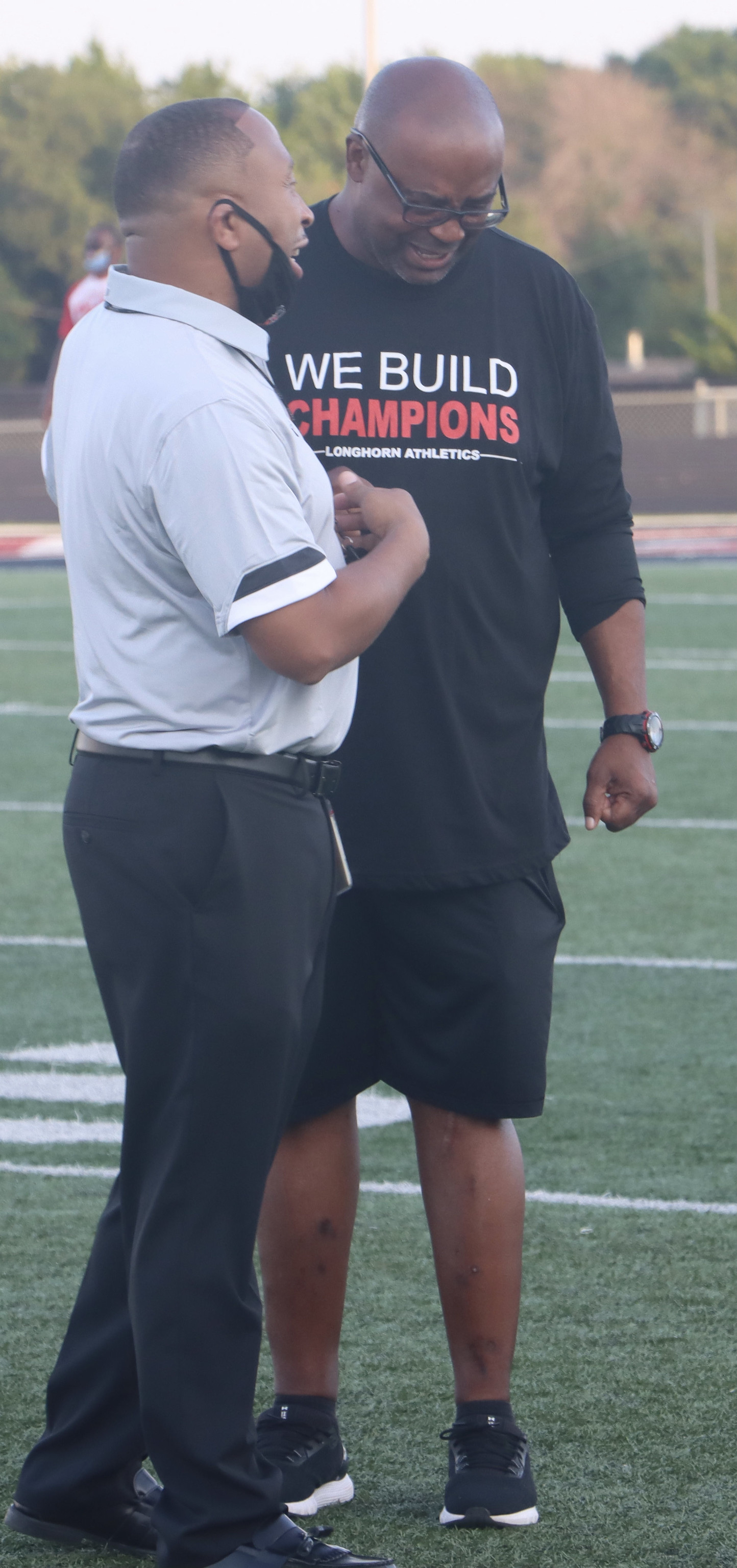On a sunny day, two African-American men stand on a well-mown green football field, featuring white-striped lines and numbering. The man on the right, who is bald or has a shaved head, is wearing glasses, a black t-shirt adorned with the text "We Build Champions" in red and white, black shorts, black and white tennis shoes with black socks, and a wristwatch on his left hand. He exudes an authoritative aura, likely indicating his role as a coach. The other man, positioned to the left and facing sideways, has a short buzzed haircut and wears a light blue shirt with a black and white stripe on the arm, black pants, black shoes, and a black face mask pulled down to his chin. This man could be a referee or another coach. Behind them, the sky is clear, and there are green trees, possibly a glimpse of the end zone, bleachers, or other structures in the background.